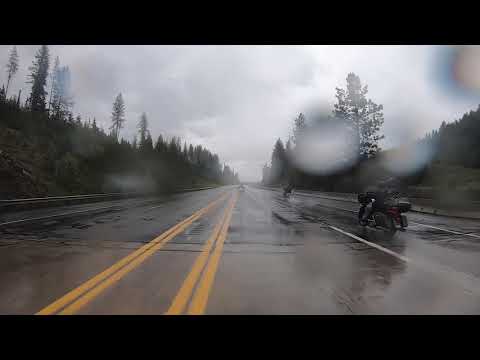The image captures a rainy scene taken from a vehicle on a wide highway, the view slightly obscured by water droplets on the lens. The sky is overcast with dark gray, heavy clouds. The wet road is divided by two sets of double yellow lines down the center, indicating no passing. To the right side, a white dashed line separates the two lanes, while on the left side, it seems to be a single lane bordered by a solid white line. Guardrails line both sides of the road, flanked by grassy hills with some shrubbery and evergreen trees. Visible through the rain, three motorcycles can be seen on the road, adding to the sense of movement in otherwise dreary weather conditions.